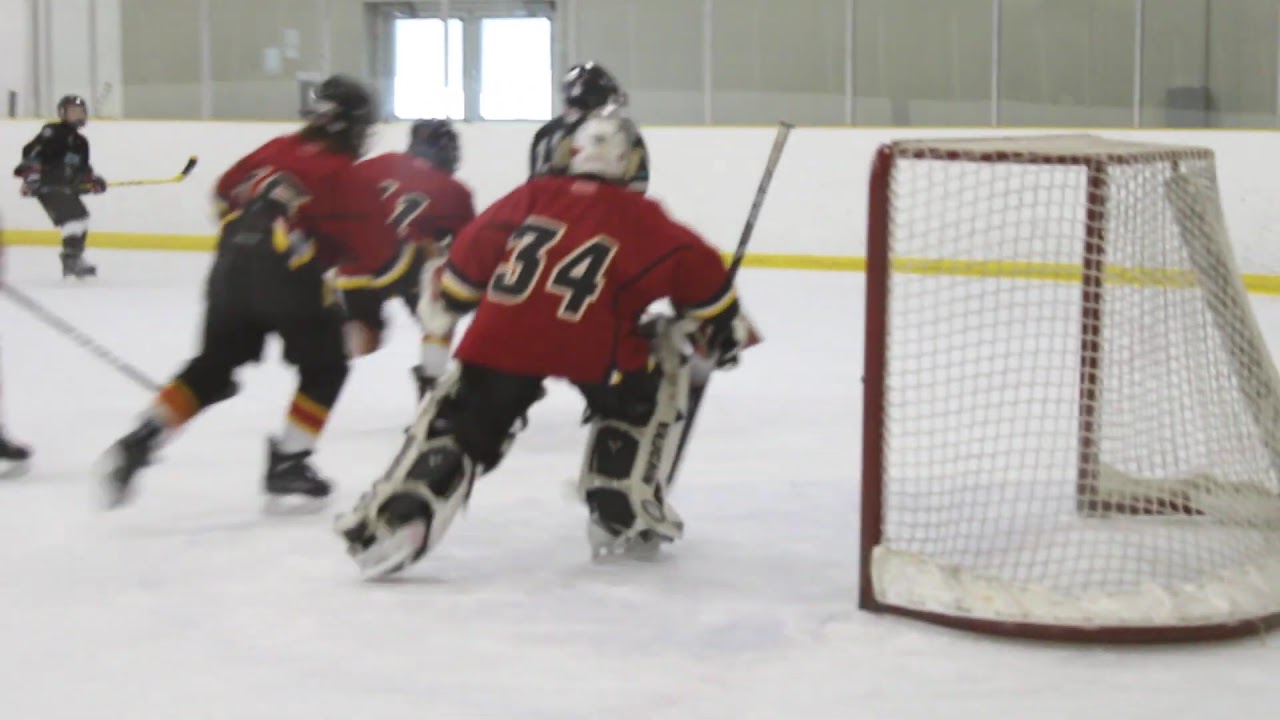The image captures an intense moment during a live ice hockey match, focusing on action near one of the goals. Prominently in the center, a player in a red jersey with the number 34 on his back, identified as the goalkeeper, is slightly crouched, poised to defend the net. He wears a white helmet and standard protective gear, including knee guards and skates. To his left, two teammates in red jerseys, numbered 16 and 11, skate towards players from the opposing team. Closest to the camera, another player in red moves across the ice. On the periphery, two players from the opposing team, dressed in black uniforms, are also visible. One of these opposing players is directly in front of the goalkeeper, while another can be seen in the top left corner, holding his hockey stick aloft. The action takes place on a white ice rink surrounded by a white barrier and transparent plastic screens. In the background, beyond the glass, a door and windows are visible on the top left. Additionally, an unidentified skate near the frame's left edge hints at more off-screen action.